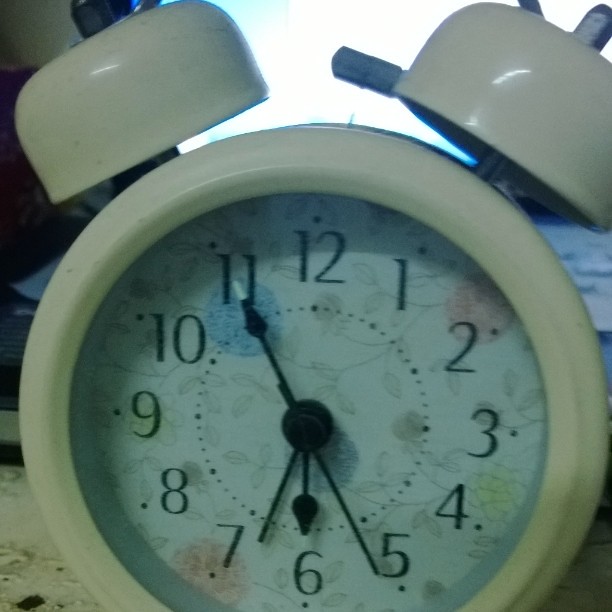This is a close-up color photograph of an old-fashioned, white alarm clock with a smooth, curved body and two white bells connected by a spring on top. The clock face features a white background adorned with a repeating pattern of petite flowers, in shades of blue, pink, and yellow, with faint green vines that create a delicate, interconnected design. The black numbers around the clock, from 12 to 11, are arranged in a clockwise direction. The clock's black hands - the hour, minute, and second hands - point to 6:55. The clock is positioned against a bright white background, with some blue writing on white papers visible to the right and a tan, patterned contact paper surface to the left. The background hints at sunlight streaming through a window, adding a warm glow to the scene.